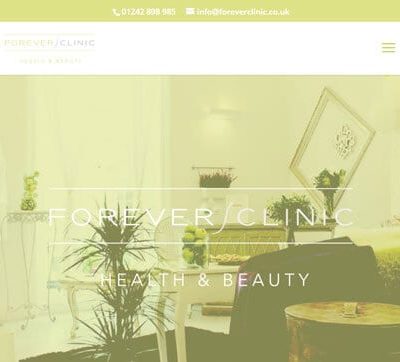The image is a screenshot of a website homepage for the business, "Forever Clinic Health and Beauty." The page features a light green and sage color scheme with white text. At the top of the image, a bar includes the company's phone number, email address, and a three-line hamburger menu for navigation. The top-left corner prominently displays the Forever Clinic logo. The main background image, tinted green, depicts a beautifully arranged room with various furnishings. Central to the layout, the clinic's name, "Forever Clinic Health and Beauty," is displayed in white letters between two horizontal lines. The room shown includes a green spiky plant with three layered spikes, a brown round wooden table, a cream-colored desk, and a crooked piece of artwork on the wall. A small table appears to have citrus fruit, possibly oranges or limes. For more information, a web address provided is www.FEMA.gov.